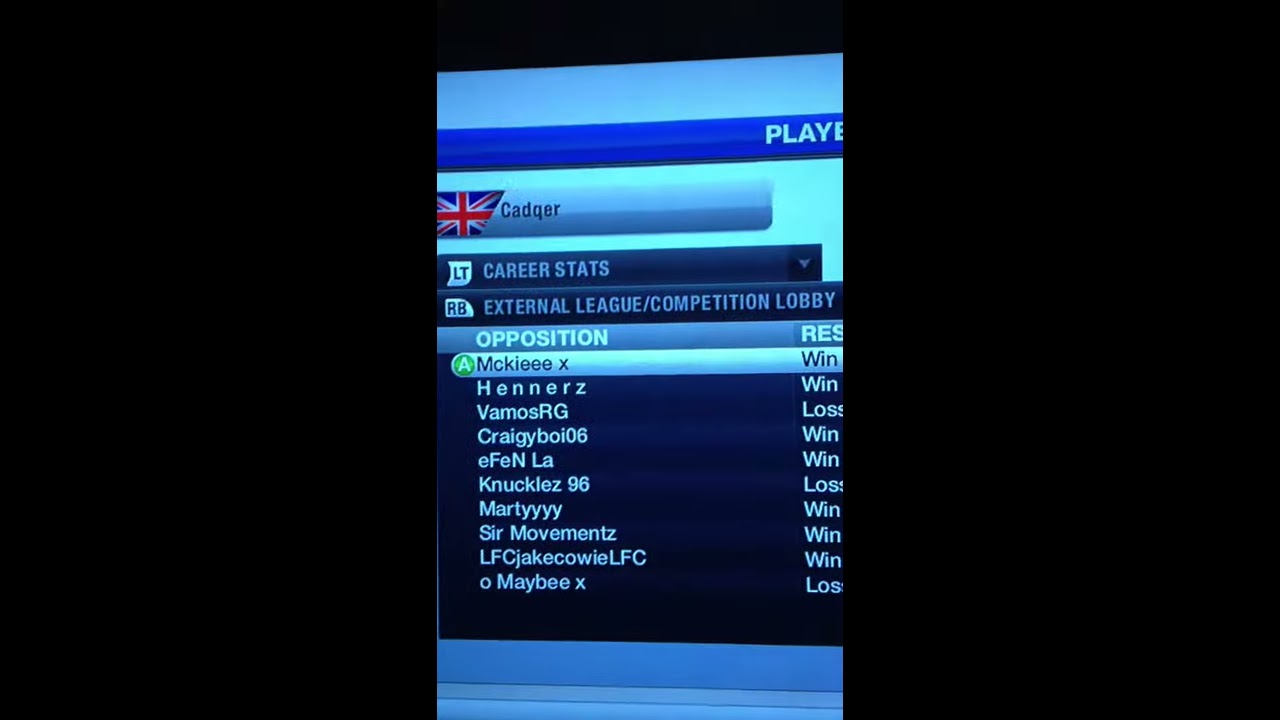This image is a detailed photograph of a sports team statistics screen, set within a larger black, three-panel frame. The central panel, slightly smaller and in portrait orientation, displays a colorful, detailed snapshot of a player scoreboard from what appears to be a competitive league, likely a fantasy or video game league. The top of the scoreboard features a partially cut-off word "PLAYER" in a blue strip. Below it, a lighter blue strip holds a Union Jack flag followed by the name "CADGER." Further down, a dark blue strip reads "career stats," and another beneath it says "external league / competition lobby."

The main section of the scoreboard, titled "opposition" in white lettering against a lighter blue background, lists the outcomes of various matches. It features about 10 team names and their corresponding results, such as:

- Vamos, RG (lost)
- Craigie, Boy, 106 (win)
- EF, EN, LA (win)
- Knuckles, 96 (lost)
- Marley (win)
- Sir, movements (win)

The scoreboard is highly detailed, capturing not only the teams and outcomes but also demonstrating the style of photographic representationalism realism, making the digital elements appear lifelike.